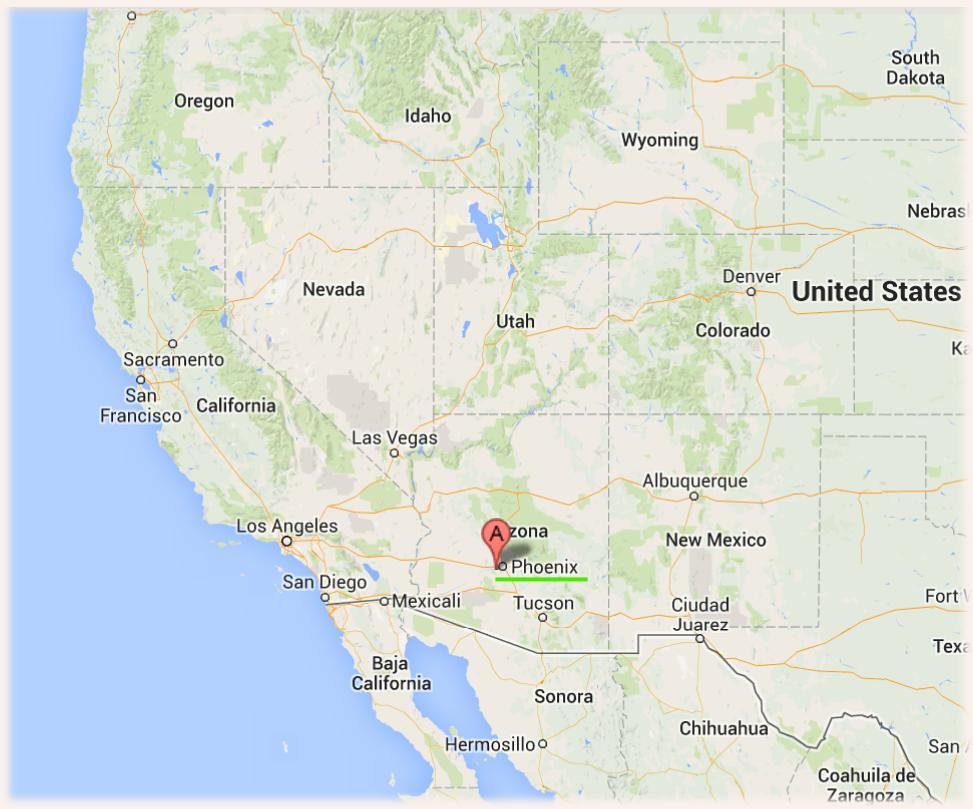This partial map of the western United States and northern Mexico, captured from Google Maps, prominently displays a red teardrop pin labeled "A" at Phoenix, Arizona. The detailed map outlines various states including Oregon, Idaho, Wyoming, South Dakota, Nebraska, Colorado, Utah, Nevada, California, Arizona, New Mexico, and Texas. Major cities such as San Diego, Los Angeles, San Francisco, Sacramento, Las Vegas, Denver, and Albuquerque are visible. At the bottom, there is a clear border line dividing the U.S. from Mexico, with northern Mexican states like Baja California, Sonora, and Chihuahua represented. Notable Mexican cities featured include Mexicali, Hermosillo, Ciudad Juarez, and Chihuahua. The map also includes topographical elements, with green-textured regions indicating mountainous areas, and a blue left edge symbolizing the ocean.